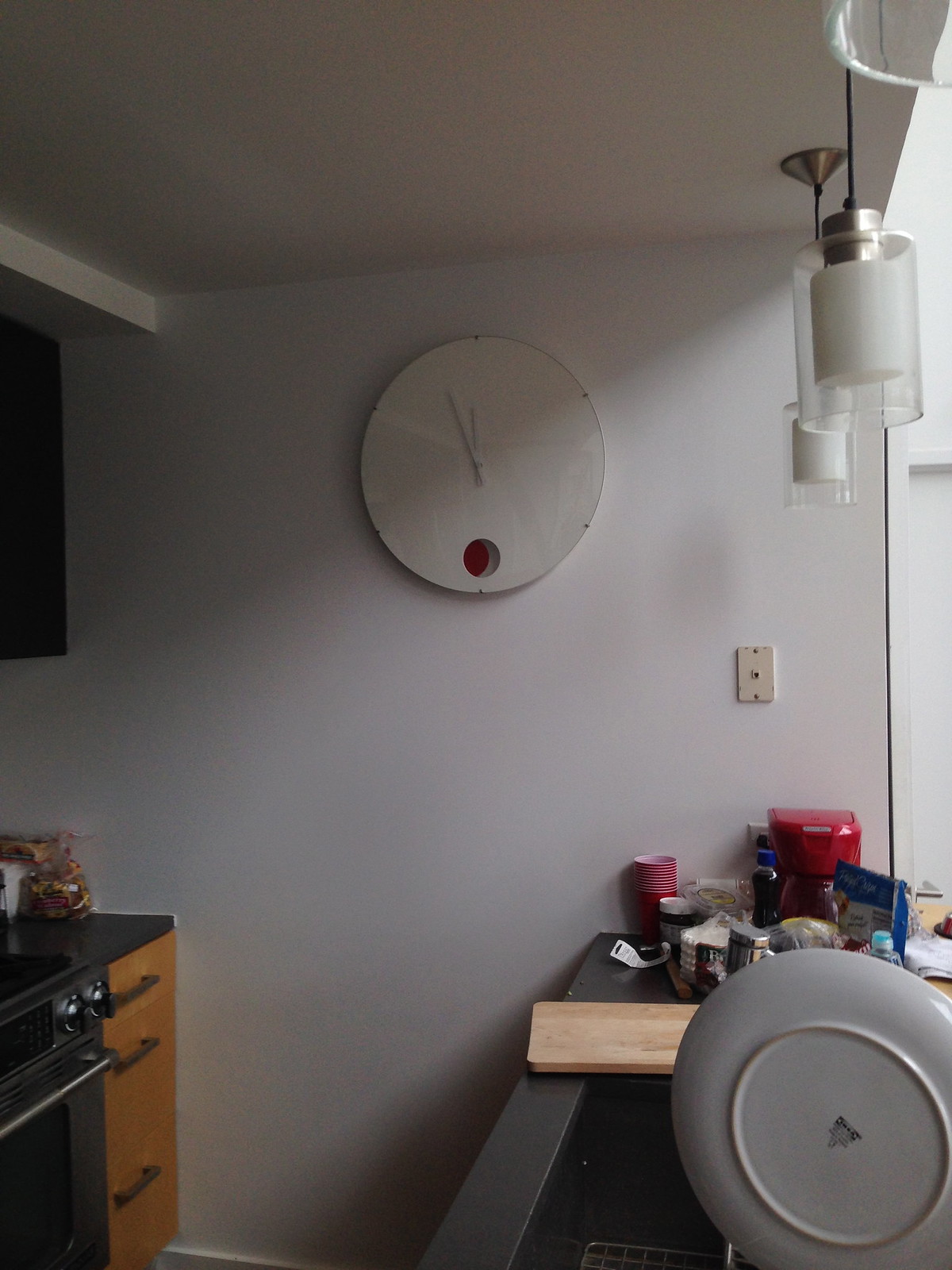The image depicts a small kitchen seen from a side perspective. Dominating the view is a stark white back wall featuring a minimalist white clock with sleek, white hands positioned around 12:55. Distinctively modern, the clock has a red semi-circle at its bottom. To the right of the clock, an old-fashioned phone plug is visible. Hanging from the flat, white ceiling are two modern light fixtures with silver bases and opaque glass covers.

Beneath the lights sits a contemporary black sink with a few clean dishes in the drying rack, including cups and a chopping board. The kitchen counter is cluttered with items, such as a red solo cup, a beer can, and other unidentifiable miscellaneous objects. Positioned across from the counter is a modern oven, characterized by its silver finish, black and silver knobs, and flanked by brown wooden cabinets with sleek steel handles. Additionally, a red coffee maker can be seen on the kitchen table top to the right, adding a splash of color to the otherwise neutral-toned space.